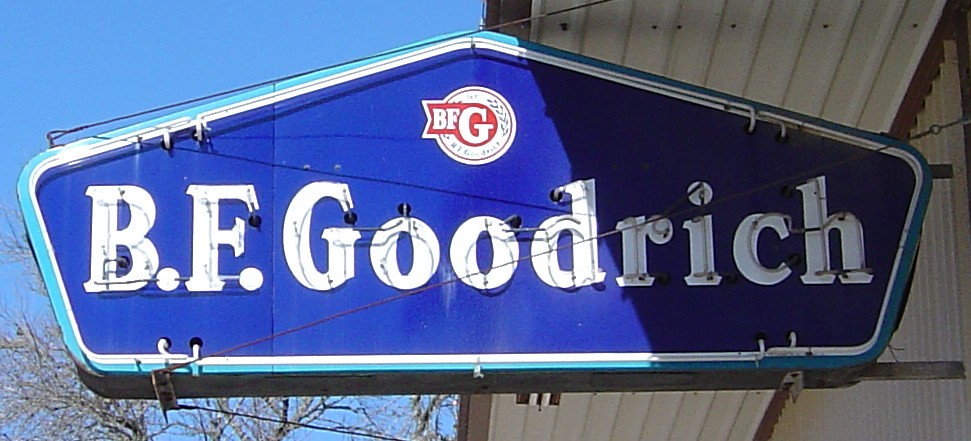This close-up photograph captures the nostalgic charm of a vintage store sign. The sign itself is crafted in the shape of a stylized house, with a horizontal base and two diagonal edges ascending outwards before curving to meet at a pointed peak, emulating a house's roof. All corners and edges are gracefully rounded, giving a softened aesthetic to the design. 

The sign features a light blue frame that encases a striking inner border of white. The majority of the sign is a vivid royal blue backdrop that prominently displays the store's name, "B.F.Goodrich," in bold white letters. Above this text sits a circular logo, displaying "BFG" in white against a rich red center. This emblem is encircled by a white band, which itself is surrounded by a thinner red line, adding a touch of intricate detailing.

The sign appears to hang just below the overhang of a corrugated white roof, indicative of traditional storefront architecture. It is sturdily attached to the building by two metal poles situated on its right side. The left side of the image opens up to reveal a clear, light blue sky and barren trees devoid of leaves, enhancing the scene with a seasonal touch. The natural elements, juxtaposed with the vintage sign, create a picturesque snapshot of Americana.